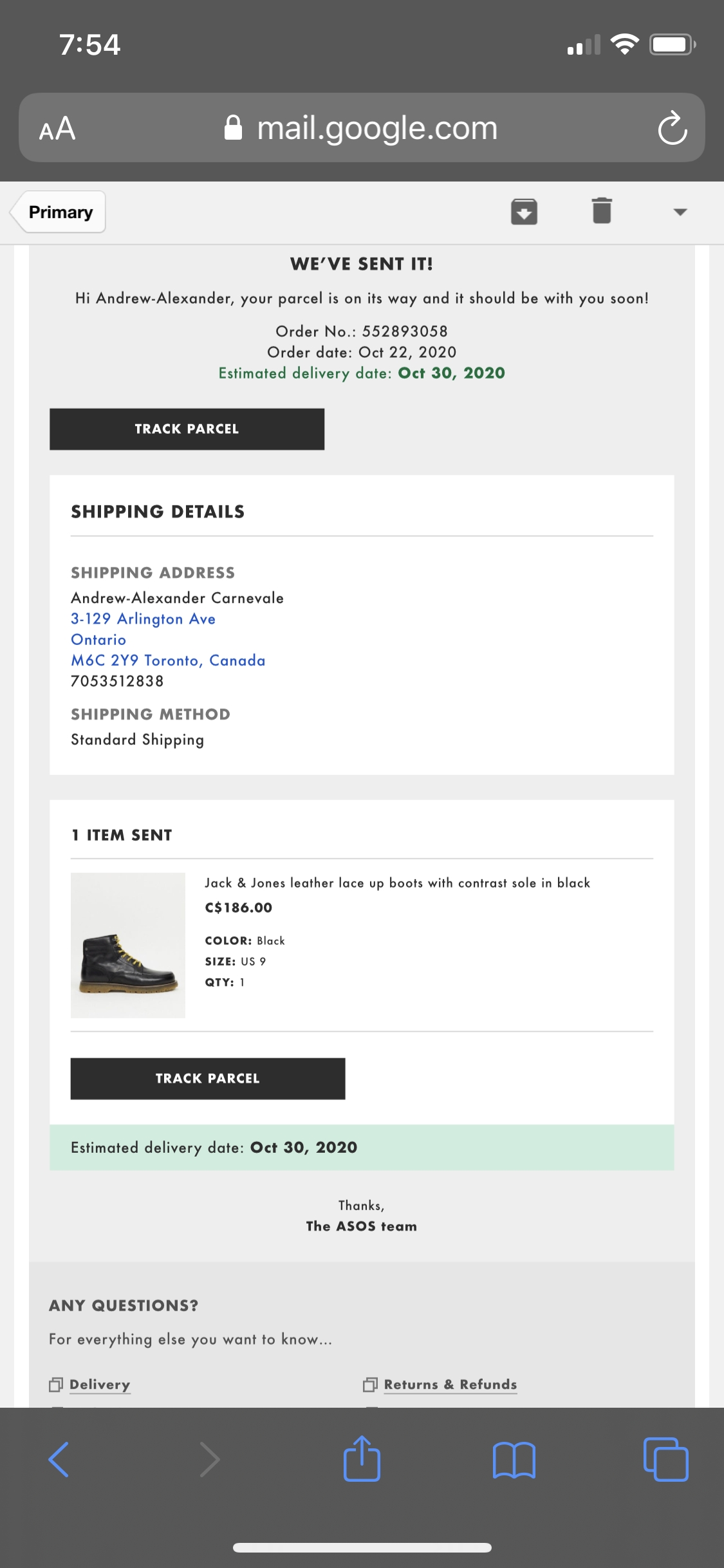This is a detailed screenshot from an iPhone's Safari browser, showing an email open in Gmail. 

**Top Status Bar:**
- **Time:** Displayed at the top left, showing 7:54.
- **Connectivity:** Two bars of service, full Wi-Fi signal, and a mostly full battery icon on the top right.

**URL Bar:**
- **Options:** Text editing option, a lock emoji indicating a secure connection.
- **Address:** mail.google.com, with a white refresh button to the right.

**Email Interface:**
- **Navigation:** An arrow to return to primary emails on the left, an option to archive the email on the right, and a trash icon for deletion.
- **Content:** 
  - **Heading:** 'We Sent It'
  - **Greeting:** "Hi Andrew, Alexander,"
  - **Message:** "Your parcel's on the way and it should be with you soon."
  - **Details:** Includes an order number and order date (October 22nd, 2020), with an estimated delivery date of October 30th, 2020, shown in green text.
  - **Button:** 'Track Parcel'

**Shipping Information:**
- **Box:** Displays shipping details, including the recipient's name, address in Toronto, Ontario, Canada, and the phone number. The shipping method is listed as standard shipping.

**Item Description:**
- **Product:** Jack and Joan's Lover lace-up boots with contrast sole in black.
- **Image:** A picture of one of the boots is shown on the left.
- **Price:** CAD 186.00
- **Details:** Color - Black, Size - US9, Quantity - 1

**Additional Information:**
- **Button:** Another 'Track Parcel' button followed by another estimated delivery date in green.
- **Closing:** "Thanks, The ASOS Team."
- **Support:** Options for questions about delivery or returns and refunds.

**Navigation Bar:**
- **Color:** Gray, located at the bottom of the screen.